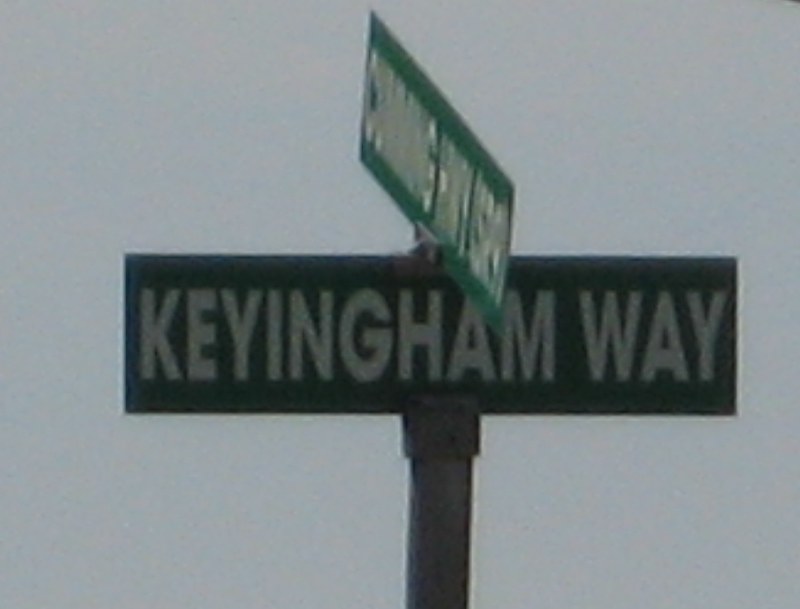The image depicts a close-up of a street sign at an intersection, taken with substantial zoom, resulting in a pixelated and grainy appearance. The photograph captures the street signs mounted on a galvanized steel post against a pale gray sky. The lower of the two green signs, with white lettering, reads "Keyingham Way" (K-E-Y-I-N-G-H-A-M Way), marking the street that runs perpendicular to the viewer's perspective. The top sign, which appears blurrier and difficult to decipher due to the angle and image quality, seems to start with a "C" and possibly contains three words. The mounting bracket securing the top sign is clearly visible.